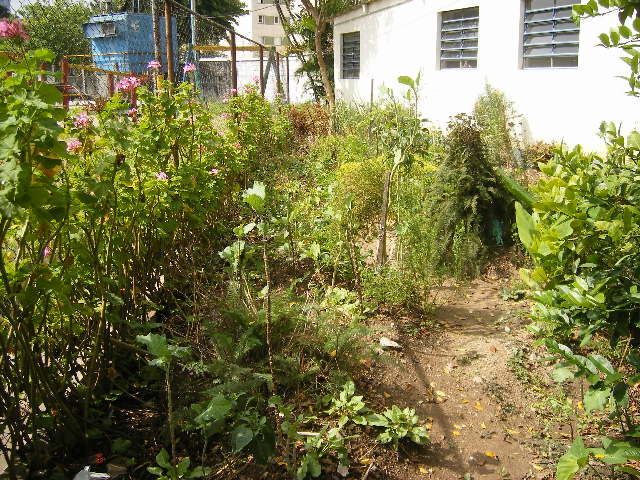This image depicts a small, somewhat dilapidated backyard adjacent to a low, white bungalow. The bungalow features three windows, each framed by six long, narrow glass panes that open and close with a wind-up mechanism. The yard itself is overgrown, with an abundance of weeds, shrubs, and patches of dirt interspersed among the greenery. Amidst this untended garden, pink blooming flowers add a splash of color. A see-through woven-wire fence runs along the perimeter of the yard, to the left of which stands a large blue structure resembling a garbage dumpster. Beyond the fence, in the distance, an apartment building and another white building are visible, adding an urban backdrop to the untamed garden scene.